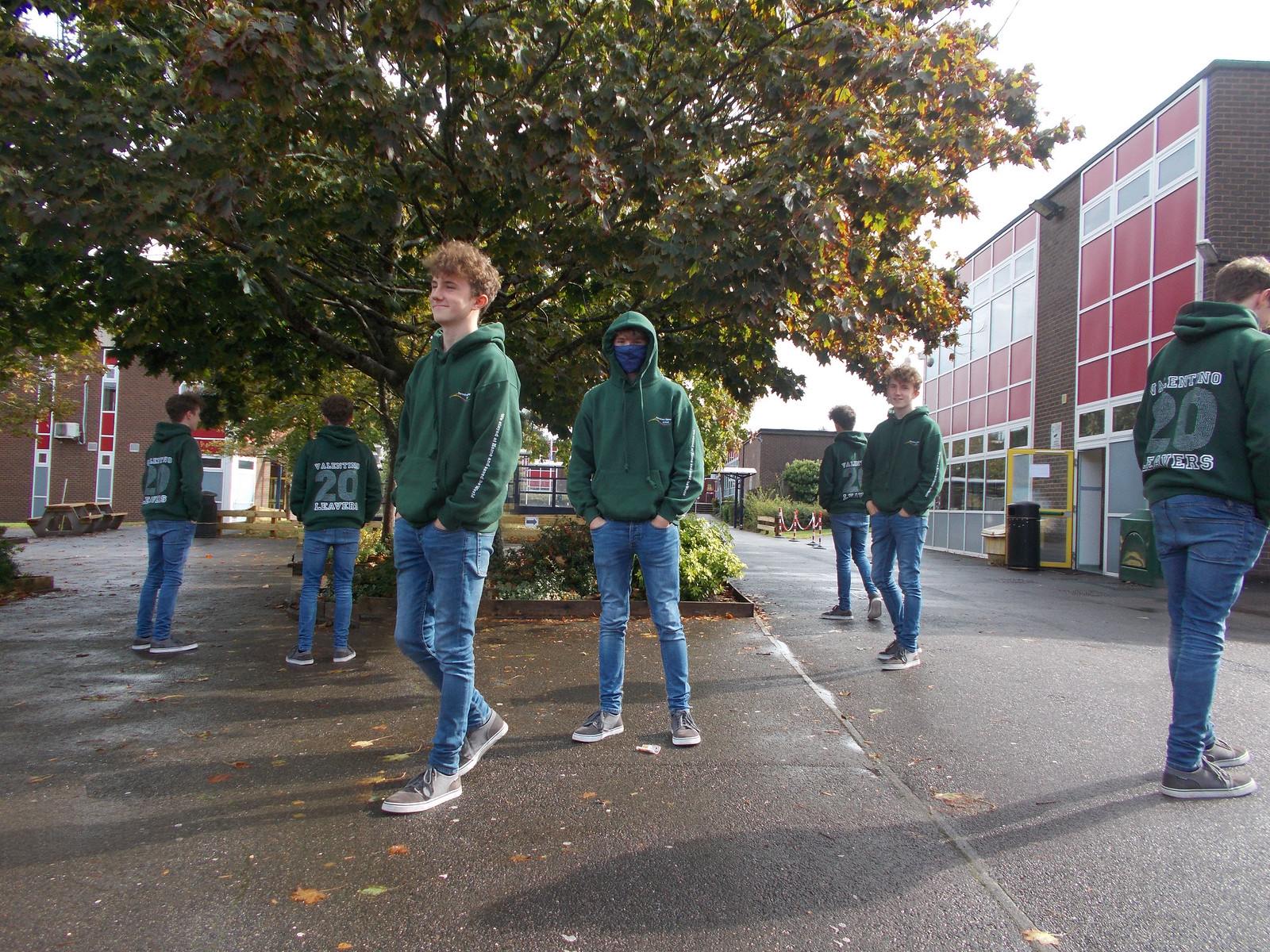In the photo, there are seven young men dressed identically in dark green hooded sweatshirts, blue jeans, and grey sneakers, with their hands in their pockets. The three men in the middle are facing the camera, with one distinctively wearing a blue face mask and his hood up. The man to the left of the masked individual has curly hair. All three have their hands in their pockets. Behind them, four men stand with their backs to the camera, each sweatshirt bearing the number 20 in gray and the text "Valentino Leavers" in white. The setting appears to be an outdoor campus area with asphalt ground, a large prominent tree, and a red and gray building to the right in the background, along with another brown structure on the left. It is daytime with an overcast sky.